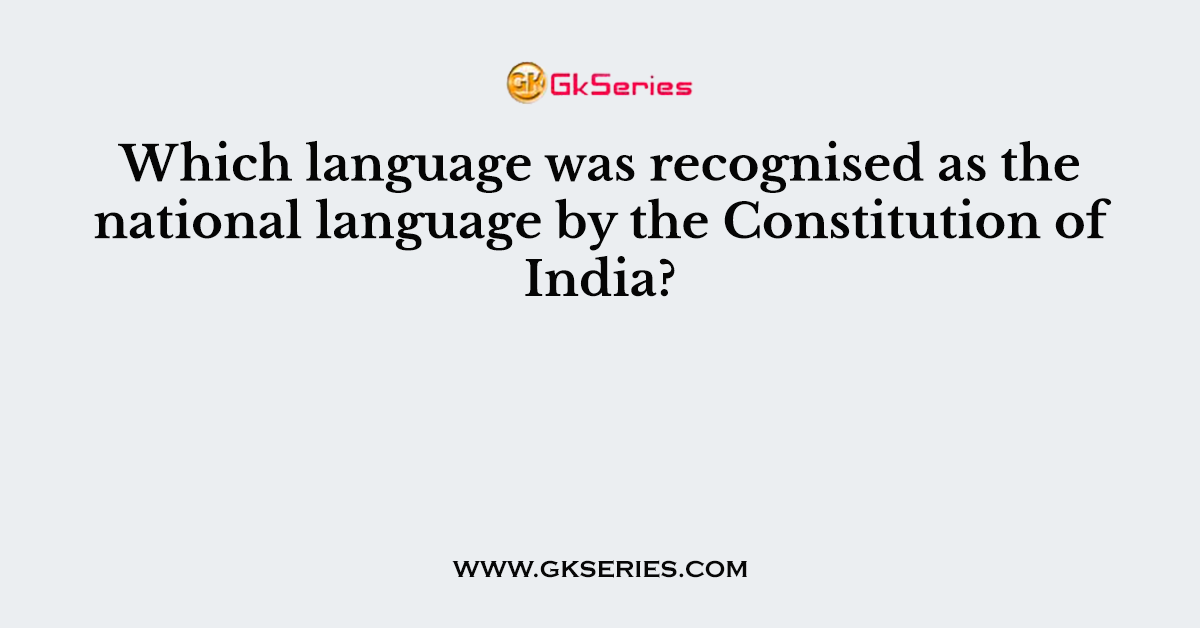This rectangular graphic features a solid gray background. At the very top, there is an orange and yellow circular emblem with embossed orange initials "G K". To the right of the emblem, bold red text reads "GK Series". Below this header, a central question is displayed in bold black lettering: "Which language was recognized as the national language by the Constitution of India?". This text is centered within the image. At the bottom center, a URL is displayed in black, reading "www.gkseries.com". The overall design appears to be neutral, making it unclear whether this graphic is for an advertisement, a website banner, a poster, or another medium. With no visible browser elements or contextual clues, it could potentially originate from various sources including digital or print platforms like magazines or subway advertisements.